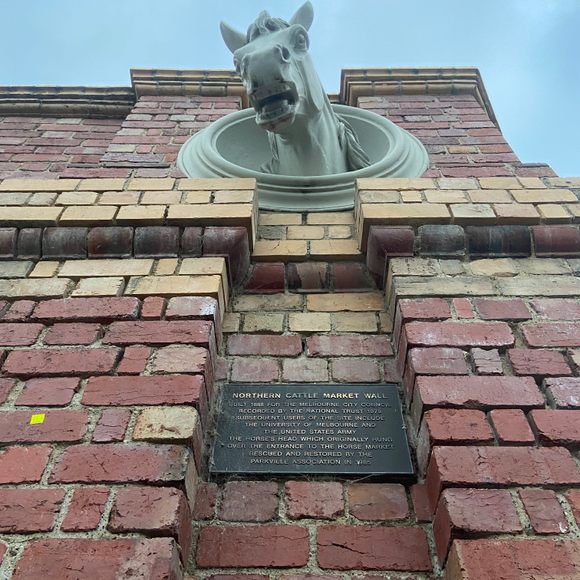The image captures a tall, weathered brick structure, likely a historical building or monument known as the Northern Cattle Market Wall. The building's brickwork features primarily red bricks mixed with occasional tan and yellow bricks, adding to its aged appearance. Midway up the wall, a prominent indentation houses a bronze plaque with embossed gold letters. The plaque, albeit difficult to read in its entirety, mentions that the wall was built for the Melbourne City Council and is recorded by the National Trust. It also makes reference to the University of Melbourne and the United States Army, and notes that the horse's head sculpture, originally hung over the entrance to the horse market, was rescued and restored by the Parkville Association. Higher up on the wall, above a ledge, a striking white horse's head sculpture protrudes. The sculpture, made of stone or marble, depicts the horse looking down with its neck and head extending from the wall, adding a dramatic and historical element to the structure. The scene is capped by a clear blue sky, offering a contrasting backdrop to the detailed brickwork and the solemn white sculpture.